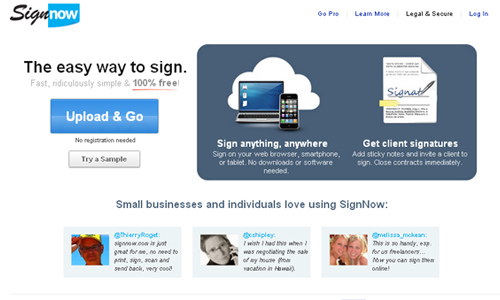This is a slightly blurry screenshot of a web page from "SignNow." In the top left corner, the logo features the word "Sign" in cursive followed by "Now" in a regular typeface, all set against a blue background behind the word "Now." On the right side of the page, there are several navigational options: "Go," "Pop," "Learn More," "Legal and Secure," and "Login." The "Legal and Secure" option is highlighted in black, suggesting the current section being viewed.

Beneath the menu, a headline on the left side reads, "The easy way to sign: fast, ridiculously simple, and 100% free." Below this, there is a blue button labeled "Upload and Go, no registration needed," and a smaller, silver-gray button that says "Try a sample."

To the right, a dark gray horizontal rectangular box with rounded edges contains two sections. The left section shows an image of a laptop and smartphone with a cloud in the background, symbolizing cloud-based functionality. Text below the image reads, "Sign anything anywhere, sign on to your web browser, smartphone, or tablet, no downloads or software needed."

The right section features an image of a document with accompanying text: "Get client signatures, add sticky notes, and invite a client to sign. Close contracts immediately." Further down, it states, "Small businesses and individuals love using SignNow." This is followed by three different panels showcasing user pictures, usernames, and testimonials.